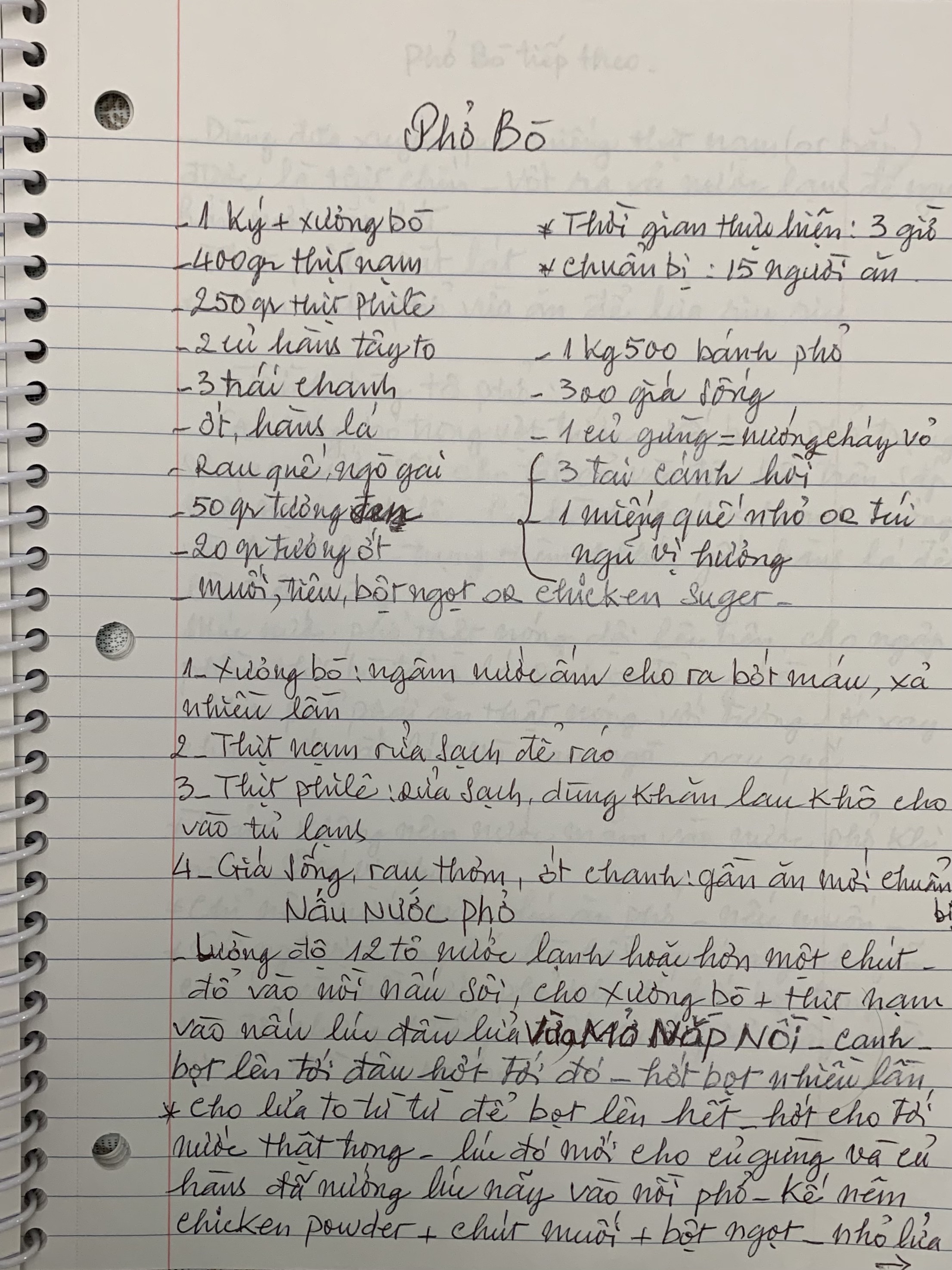The image depicts a page from a spiral notebook, characterized by its white paper with blue horizontal lines and a single red margin line on the left. The notebook is three-hole punched, and the spiral binding with white rings is visible on the left side. At the top of the page, there's a handwritten title that reads "PHO BO" or "FOBO," written in black ink in cursive. The majority of the page is densely filled with handwritten text, also in black ink, which is not in English but appears to be a foreign language that uses the Latin alphabet, possibly Vietnamese. The content seems to be a recipe, given the structured format with bullet points or numbered steps outlining ingredients and instructions. Notably, there are gaps with two blank lines above the bottom line, which is customary left unwritten. The handwriting varies in clarity, suggesting it was written quickly.